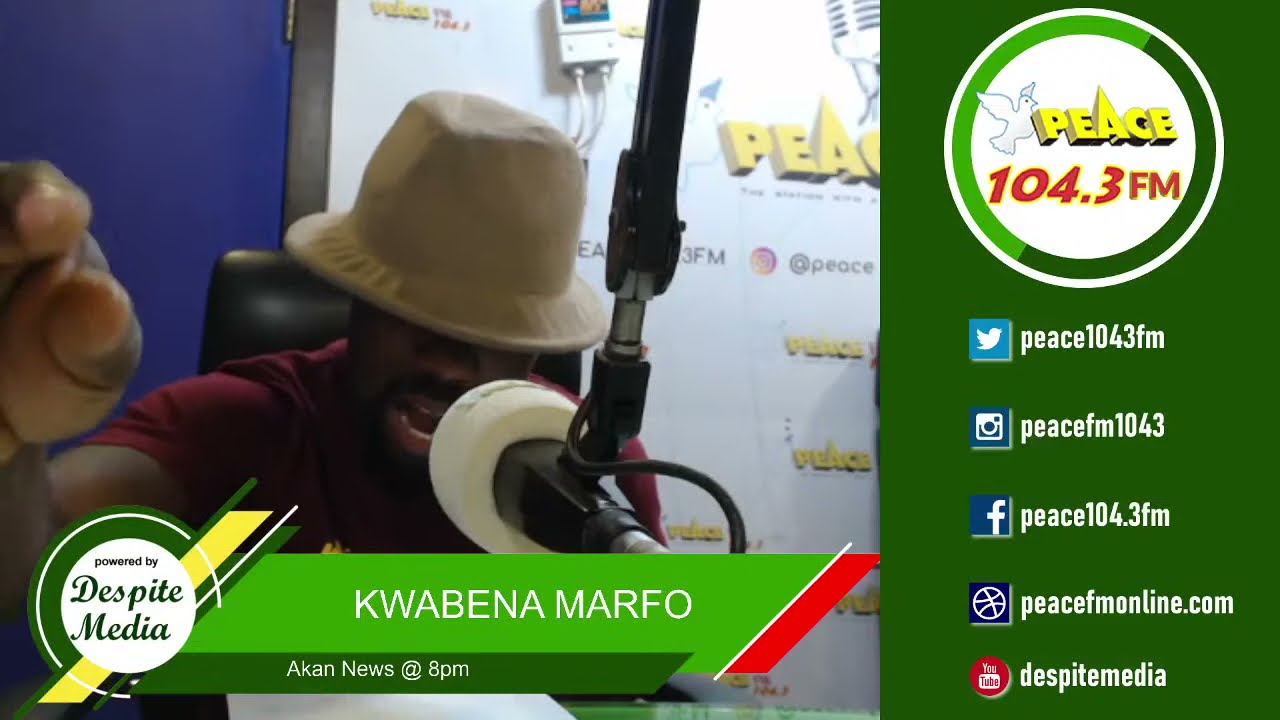The image appears to be a screenshot from a live-streamed radio broadcast featuring an African-American man named Kwabena Marfo. He is wearing a beige fedora hat that slightly obscures his eyes, and he is dressed in a purple shirt. He is animatedly speaking into a large white-cushioned microphone that hangs in front of him. Behind him, a blue wall is partially covered by a framed plaque. 

At the bottom of the image, there is a banner that reads "Powered by Despite Media," and another overlay displays "ACAN News at 8 p.m." along with Kwabena Marfo's name. The right side of the image includes a green and red rectangular graphic containing the text "Peace 104.3 FM," accompanied by the station's logo, which features a yellow italicized "Peace" with a pyramid-like 'A,' red "104.3 FM" lettering, and a dove inside a white circle with a green border. The image also provides the station's social media handles for Twitter, Instagram, Facebook, and YouTube, and mentions a website, peacefmonline.com. Kwabena Marfo is gesturing with his hands as he speaks, enhancing his expressive communication style during what appears to be a live radio talk show.